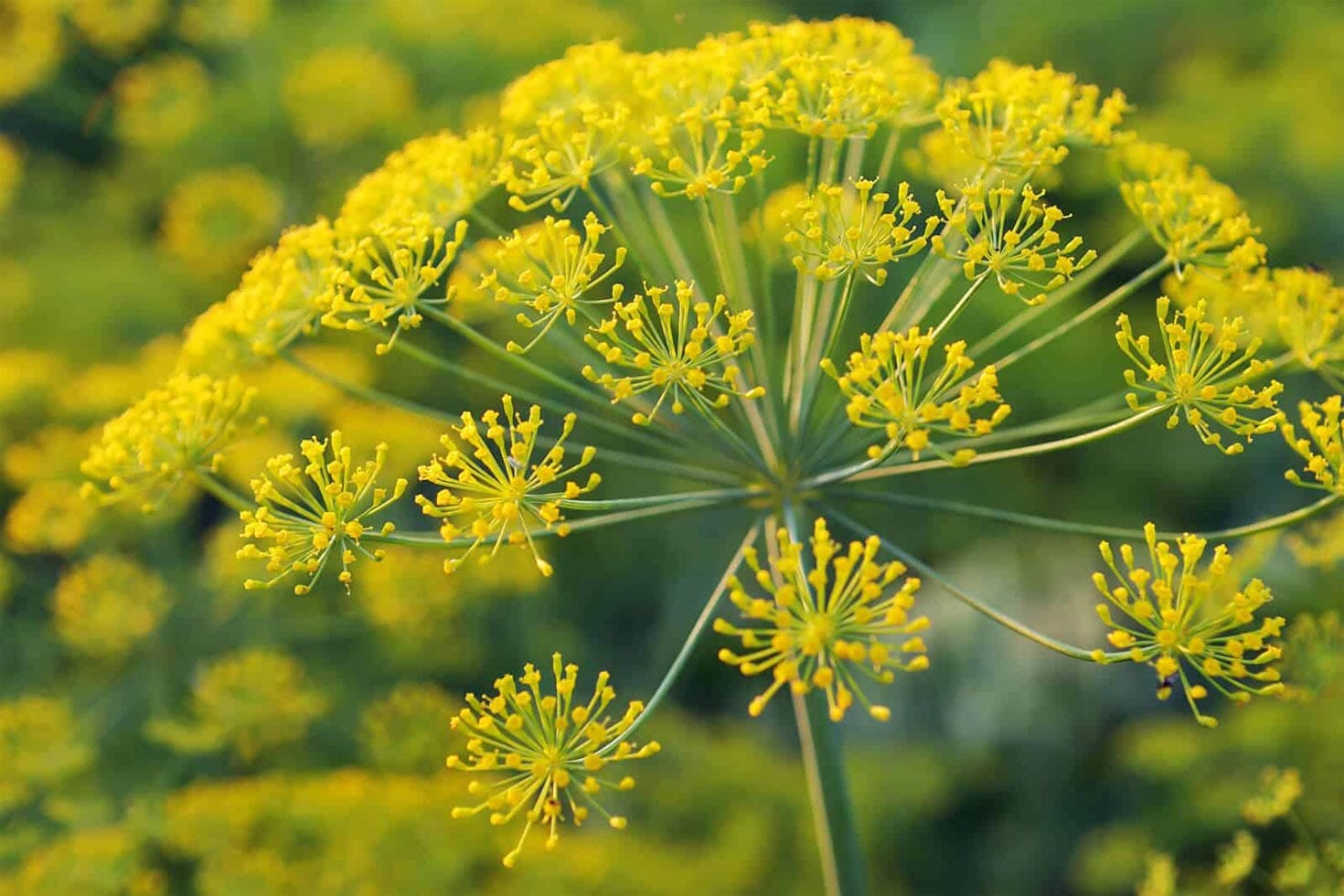The photograph captures a close-up of a delicate flowering plant taken outdoors during daytime, though the exact time is indeterminate due to the absence of visible sunlight. The main subject is a green stalk which extends into multiple thin green stems, each terminating in clusters of yellow-tipped protrusions that resemble small yellow balls. These yellow-ended branches give the plant a delicate, almost fireworks-like appearance. In the background, which is out of focus, there are numerous repetitions of the same flowering plant, creating a sea of green and yellow hues that subtly blend together. The overall composition and colors of the image evoke the sense of an expansive garden filled with these unique flowers.